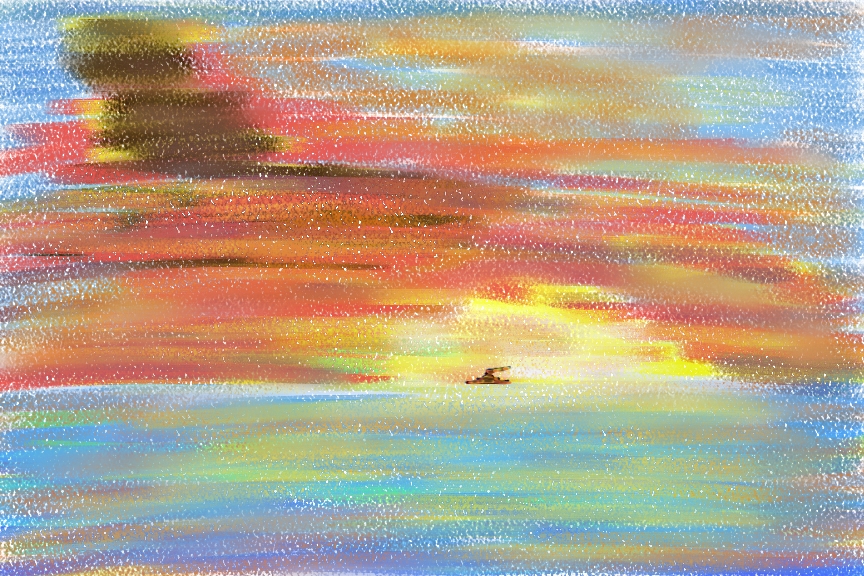The image is a vivid and colorful painting or drawing, characterized by broad horizontal brush strokes that span the entire rectangular canvas. Dominated by a sunset theme, the painting exhibits a yellowish semicircle near the center, suggesting a setting sun. Surrounding this sun are radiating streaks of reds, oranges, and touches of pink, creating a vibrant sky. Towards the top, the colors transition into a lighter blue, representing the upper sky. Below the horizon, there is a darker blue area, resembling a body of water, which reflects the colorful streaks from above, including some yellow and faint green hues near the sun’s reflection. The painting also features a small, unclear brown or black object near the center and another indistinct black streak in the upper left corner. The entire composition utilizes brush strokes that predominantly move left to right, creating a harmonious blend of colors throughout the scene.